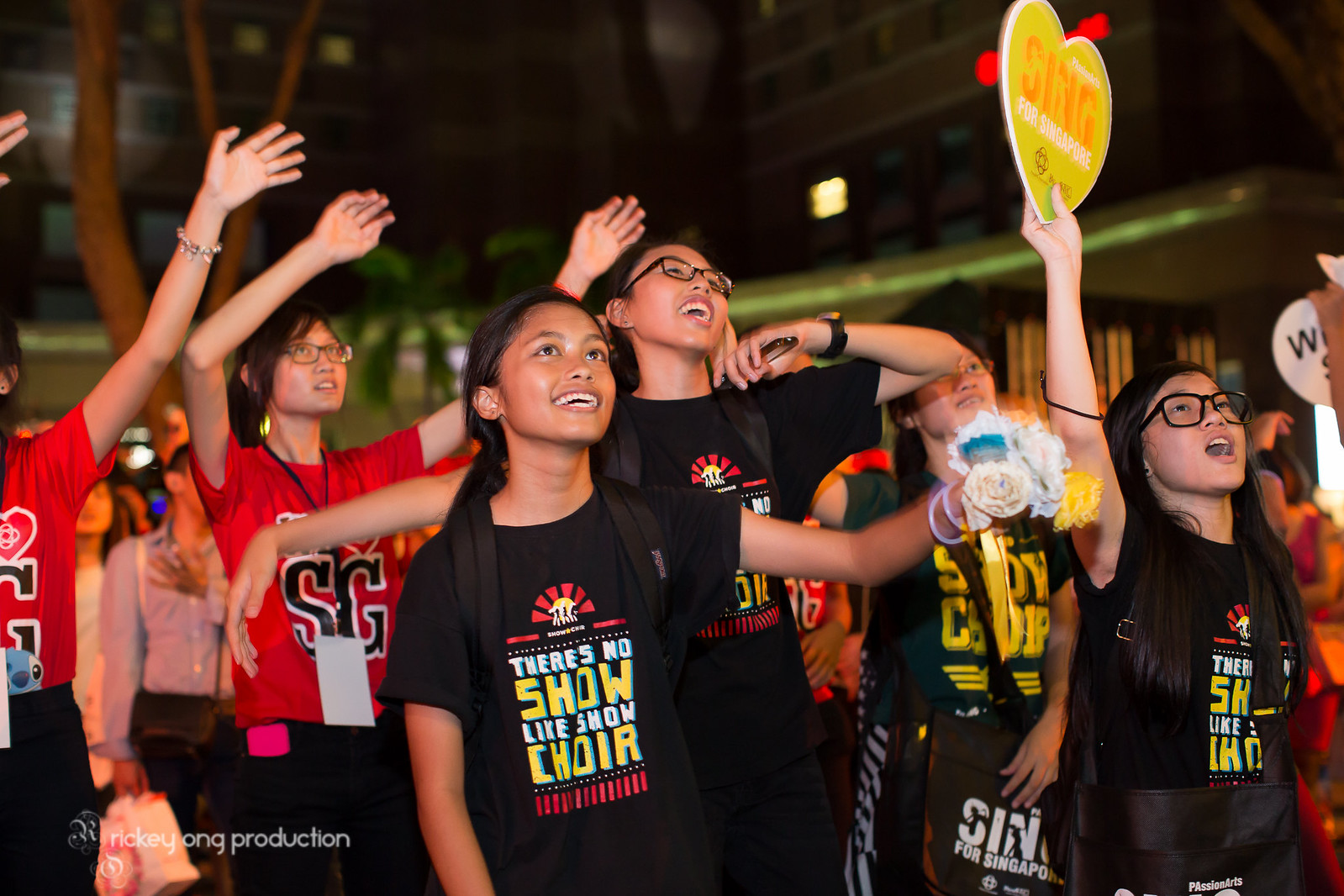In this color photograph, captured at night in landscape orientation, we observe a vibrant outdoor scene dominated by a diverse crowd of enthusiastic young people. Against a backdrop of dark skies and dimly lit buildings, the foreground features four smiling Asian teenagers standing at the center, dressed in matching black t-shirts with a bold red, white, and yellow graphic that reads "There's no show like show choir." They gaze and cheer towards something out of view on the top right, emitting a sense of communal excitement.

Surrounding them are more young individuals, some clad in red jerseys emblazoned with the letters "SG" in black and a heart symbol, further contributing to the lively atmosphere. A few of the participants hold signs and roses, with one notable heart-shaped sign bearing the words "Sing for Singapore" in gold and red, enhancing the impression of a celebratory event or concert. 

The overall setting is partially illuminated with sporadic lighting that reveals elements like green-lit palm trees and other urban features, leaving much of the environment shrouded in nighttime darkness. The text “Rookie Ong Production” in the bottom left corner hints at a formal event organization, rounding off this dynamic and spirited snapshot.